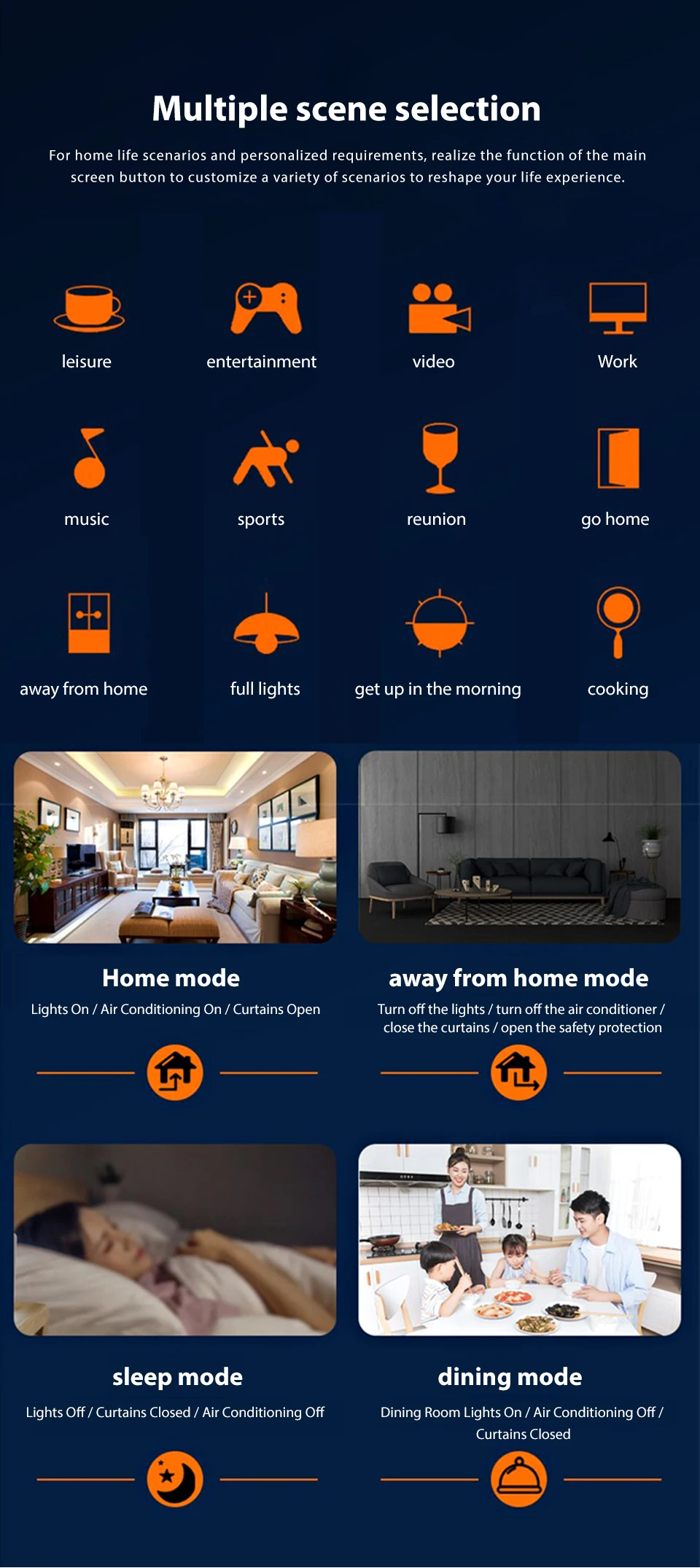This photograph resembles an informational leaflet for a smart lighting device. The leaflet features a navy blue background with prominent white font at the top, followed by smaller white text below. It presents a series of orange icons with white labels beneath each. The icons depict various items including a coffee cup, music note, window, video game controller, a person leaning with a spear, light fixture, video camera, wine glass, sun, TV, door, and skillet.

Below the icons, there are four distinct images:

1. A living room with tan walls and light-colored furniture, 
2. A setting featuring a gray wall and gray couch,
3. A woman asleep on light-colored bedding,
4. A family in a kitchen.

Each of these images is accompanied by orange icons and descriptive white text underneath, providing context for how the smart lighting can be utilized in different scenarios.